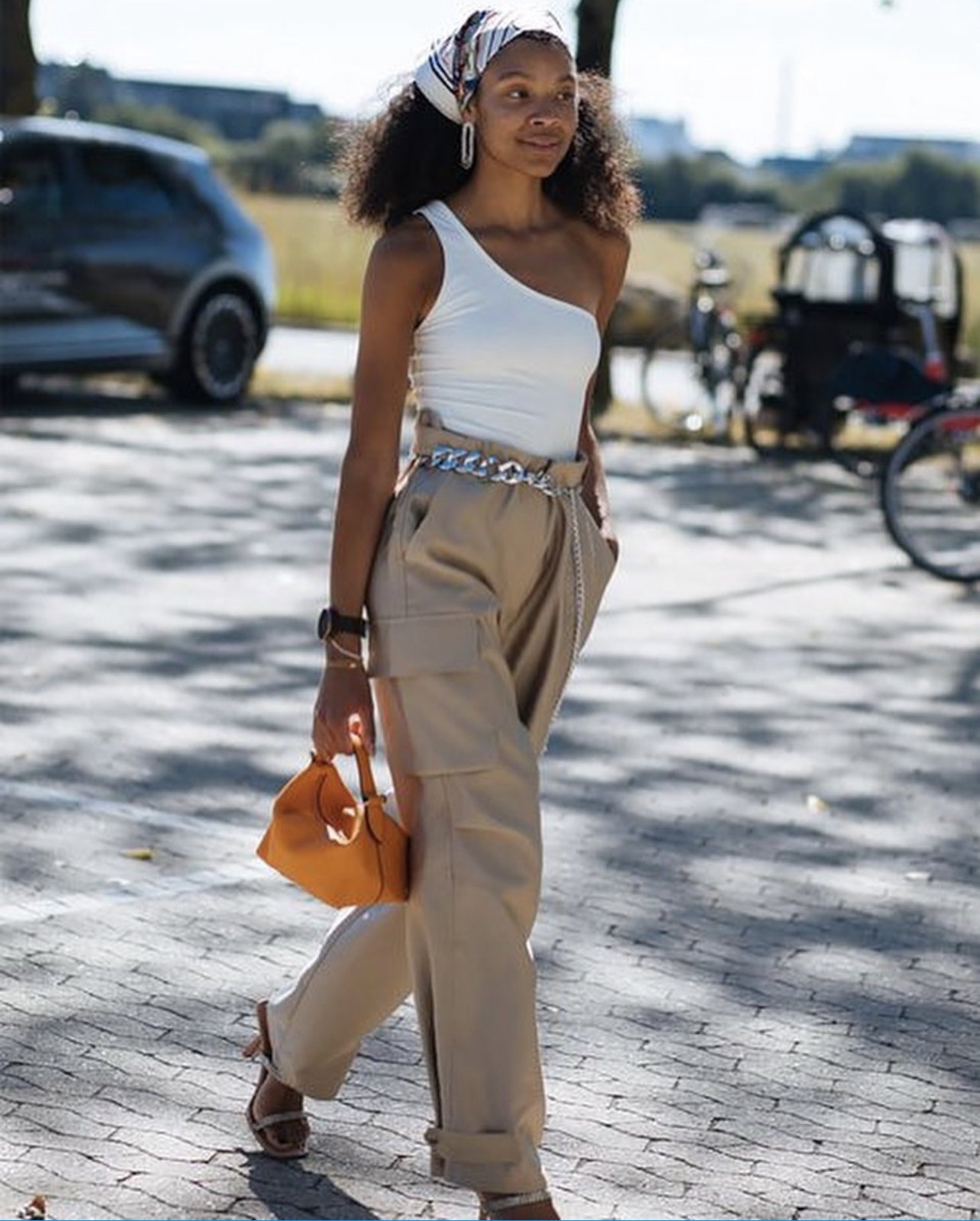The image features a young, attractive African-American woman walking on a gray stone path that resembles a fashion ad. Her long, brown, curly hair is elegantly styled with a brown and white bandana, and she has striking long silver rectangular hoop earrings. She is dressed in a chic white off-the-shoulder tank top, paired with tan paper bag pants that are cinched at the waist with a silver belt and rolled up to mid-calf. She completes the look with stylish high-heeled strappy sandals. In her left hand, she carries a bright orange satchel purse, and her wrists are adorned with a black watch and a gold bracelet. The background reveals a blurred car and bicycles alongside some buildings, suggesting an urban setting.